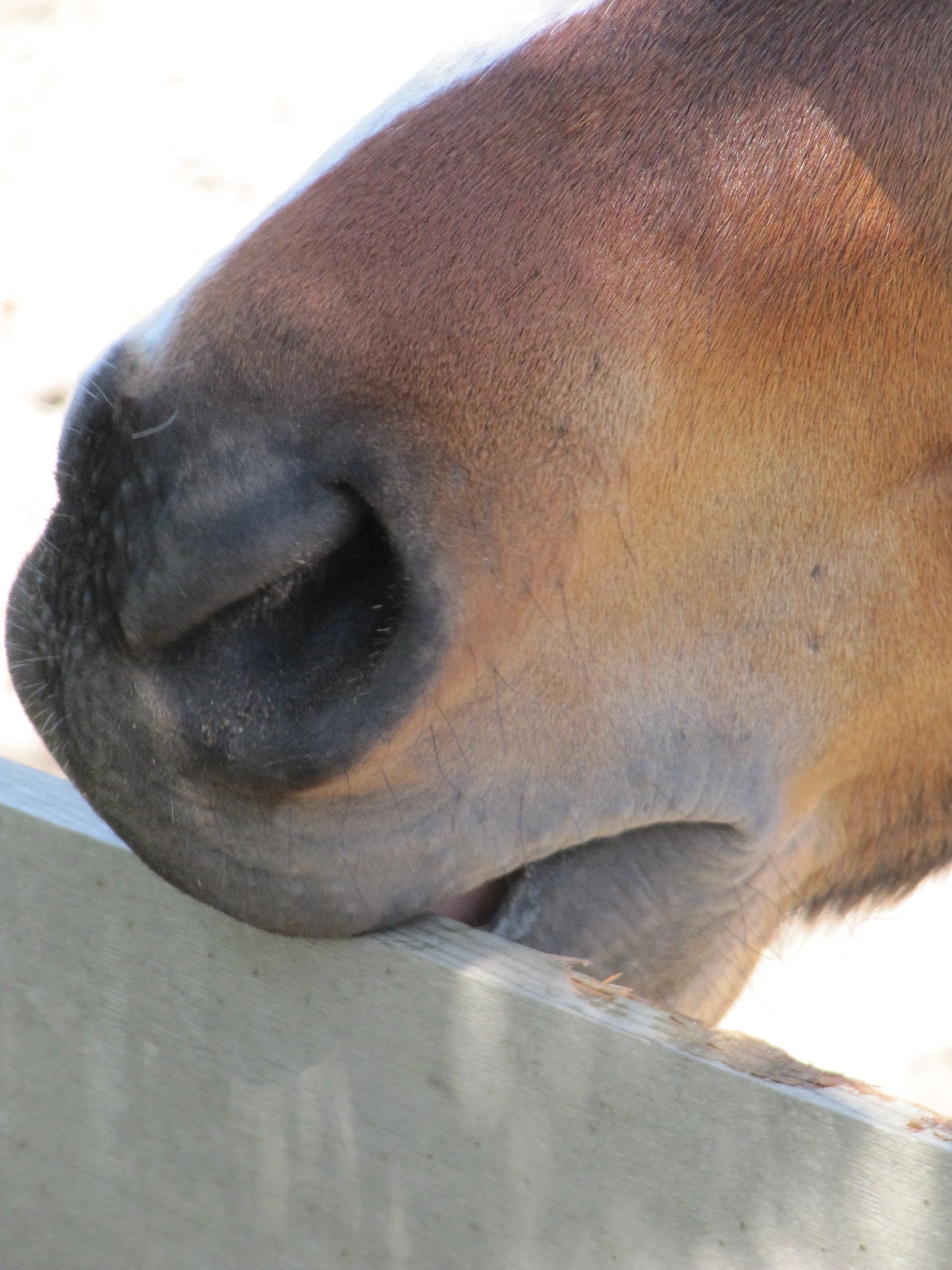The image is an up-close shot of a horse’s snout and mouth. The horse has light brown fur with a slightly darker ridge along its nose and a distinctive white stripe on top. The nose is oblong and black, resembling the entrance of a cave. The horse appears to be chewing on a wooden fence post, which shows signs of wear with chunks missing and bite marks. The fence is mostly gray from being worn down over time, but the freshly chewed parts are brown. The background is white, washed out by the sunlight. You can see only a few inches down the snout, and there is darker hair under the chin. Overall, the focus is on the horse’s chewing activity and the detailed textures of its nose, mouth, and the wooden fence.